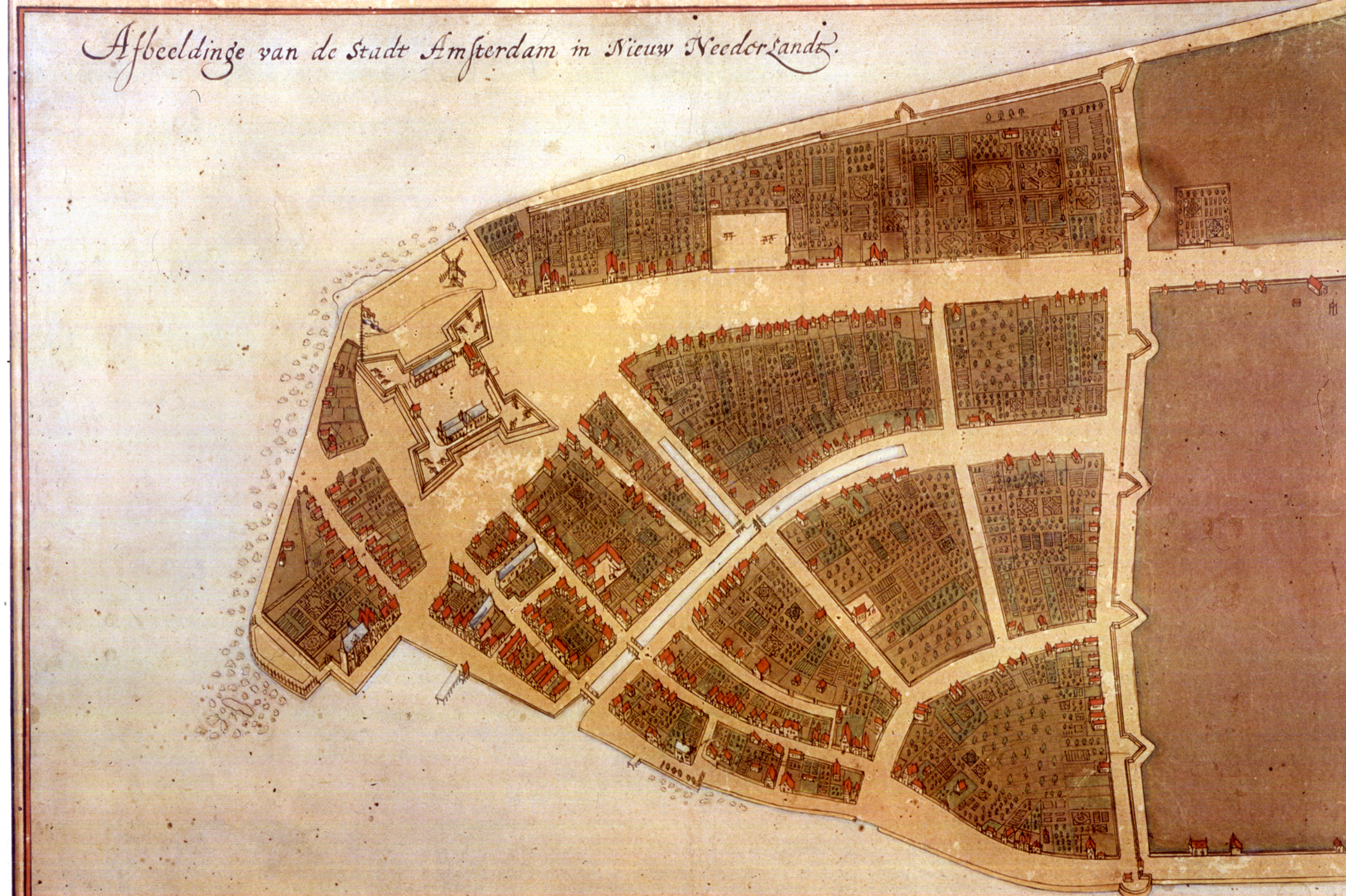The image is a detailed rectangular map highlighting a specific section of Amsterdam. Prominently, at the top of the map, some Dutch text can be seen, with the word "Amsterdam" clearly identifiable amidst it. The map intricately displays various housing areas, meticulously organized in a layout that resembles a peninsula with a narrowing tip. Buildings and homes are strategically placed throughout, with calculated gaps to facilitate easy travel across different sections of the city. This meticulously planned map is a clear illustration of the population density and the systematic approach to housing and construction within this particular area. Additionally, to the right of the map, there is an expanse of undeveloped land, suggesting potential areas for future expansion.